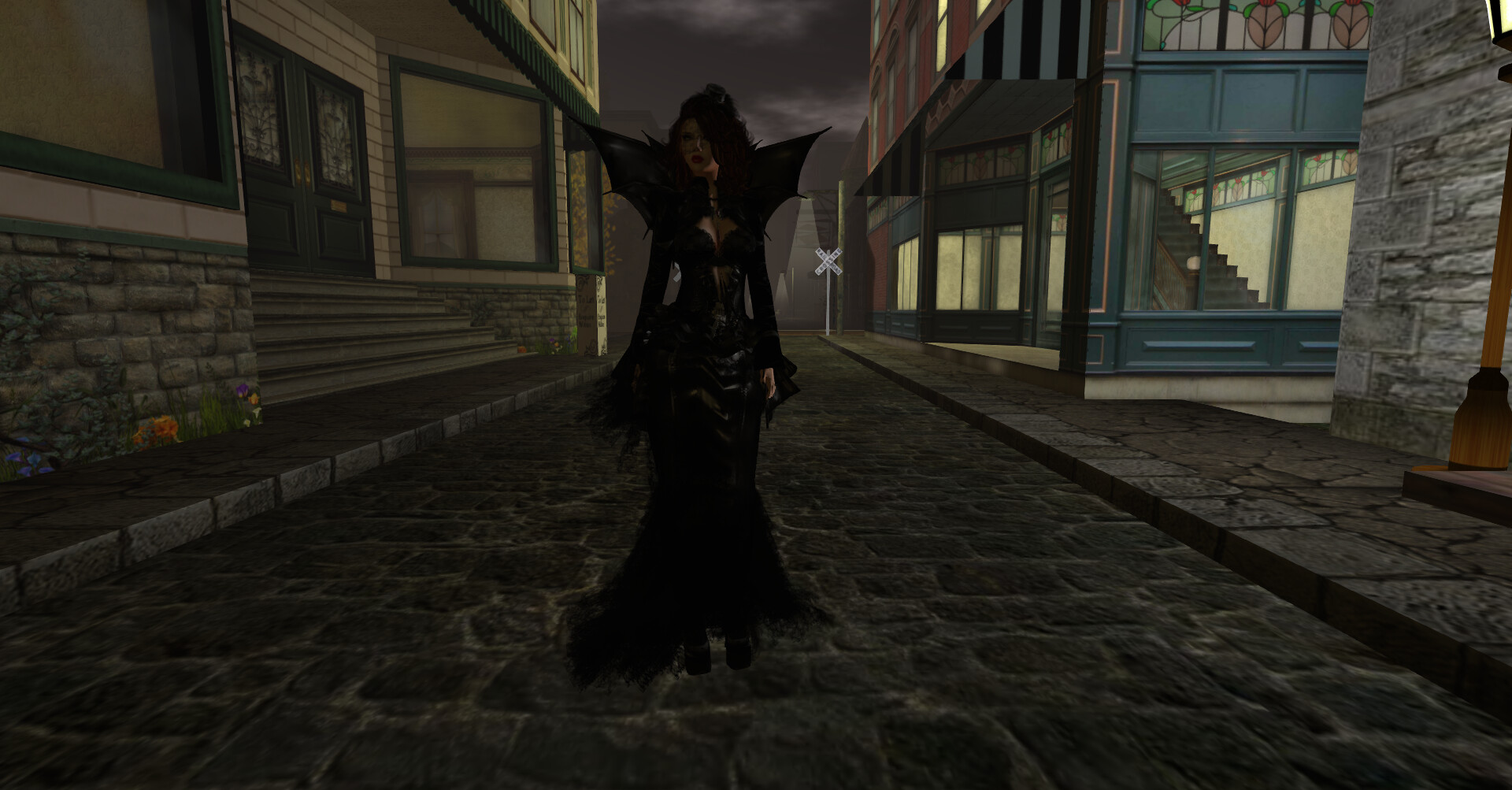The image appears to be a screenshot from a video game, featuring a female character in an elaborate, dark, and gothic costume. She stands alone in the middle of a cobblestone street, dressed in a tight, long-sleeved black gown that reaches the ground. Her dramatic appearance is accentuated by a large, vampire-esque collar that flares upwards like bat wings and dark makeup including black eye makeup and dark red lipstick. Her hair is also black with some strands hinting at purple accents. The character wears a distinctive nose piercing connected to an earring. The surrounding scene depicts an old neighborhood or cityscape, with buildings lining both sides of the stone-paved road. The buildings have a mix of architectural features, including white siding, larger stone blocks, and windows with blue and red borders. There are apparent residential or business structures with a raised sidewalk and a stone wall adorned with a few flowers. The street stretches into the distance, fading into a gray sky, with a white railroad crossing sign visible at the far end. Despite the lit street lamps and illuminated windows, the buildings seem eerily empty, enhancing the dark and solitary atmosphere of the scene.